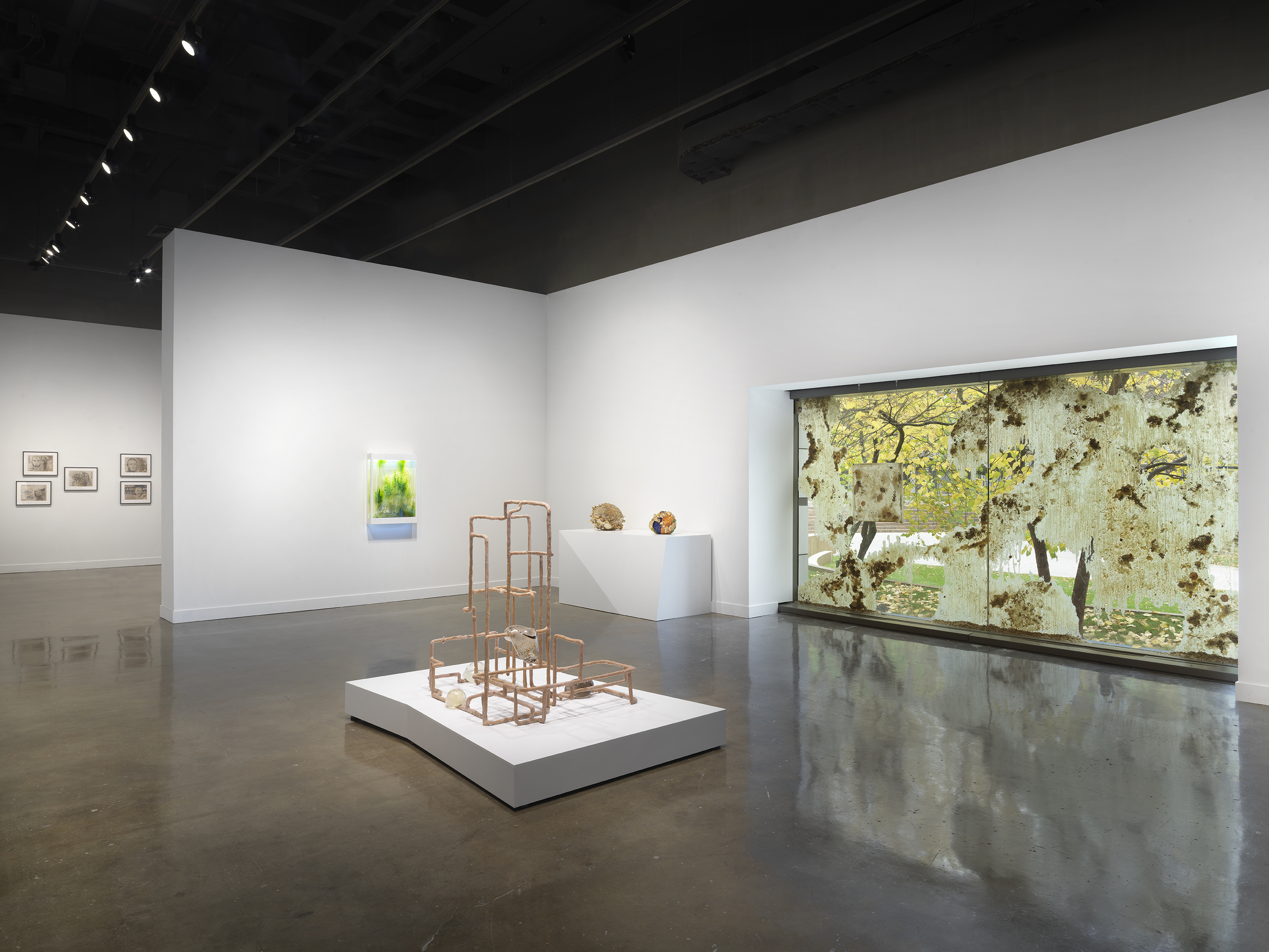This color photograph showcases the interior of a modern art museum or gallery. The ceiling is black, adorned with multiple rows of lights that illuminate the scene below. The stark white walls provide a clean backdrop for the art on display. The floor is a shiny, reflective light brown material, enhancing the room’s luminance and adding depth to the visuals. 

Dominating the space are large, wall-to-ceiling exhibits with a multitude of vibrant colors including yellow, black, brown, and green, likely indicating elaborate paintings or mixed-media installations. In the middle foreground, there’s a white platform that supports a distinctive light brown, tan structure. This structure, possibly made from metal or wood, resembles an intricate assembly of pipes, akin to a jungle gym or monkey bars.

In the background, five framed pictures are arranged—two on the left, one in the center, and two on the right—whose contents are difficult to discern. These pictures are also reflected subtly on the polished floor. Centered on a white table are two abstract sculptures: one appears to include glass with some greenery, while the other involves more complex metalwork. Together, these elements create a captivating and diverse visual experience within the gallery space.